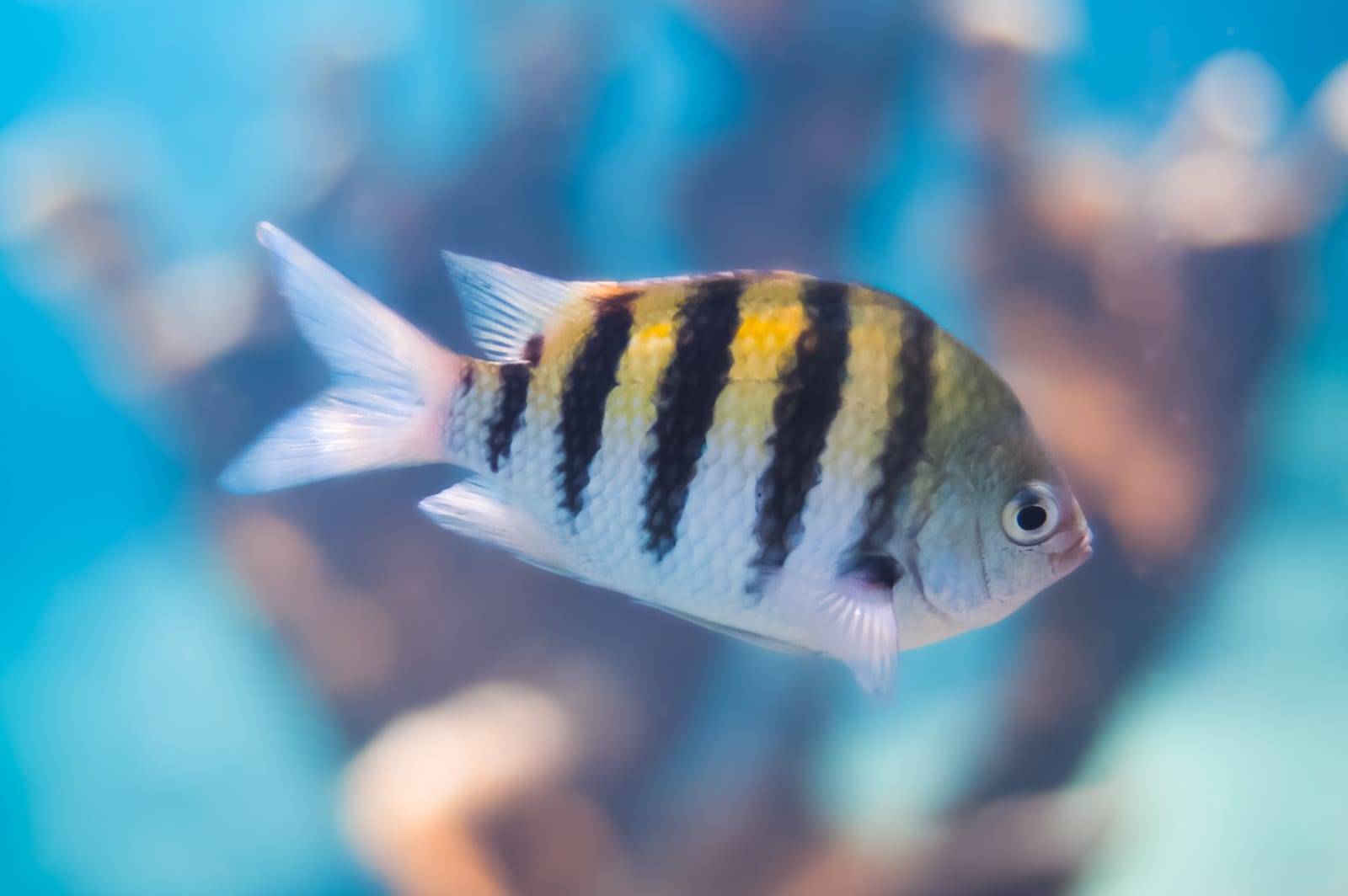This photograph captures an enchanting underwater scene centered around a single tropical fish. The fish, about the size of a sunfish, is immediately captivating with its vibrant coloration. It features a striking pattern of black stripes running down its back, interspersed with bright yellow stripes on its top half. The bottom half of the fish, including its fins and tail, is a translucent white. Its head has a subtle green tone, leading into a gray face that holds a small black eye and what appears to be a smiling expression. The background of the image is a rich blue, blending into lighter, almost white tones in some areas. Behind the fish, the backdrop consists of a blurry, brownish-orange coral reef that dominates much of the frame, along with hints of pink coral and other indistinct colorful structures. The harmonious blend of the fish's vibrant hues against the serene yet lively coral and water emphasizes the natural beauty of the underwater world.